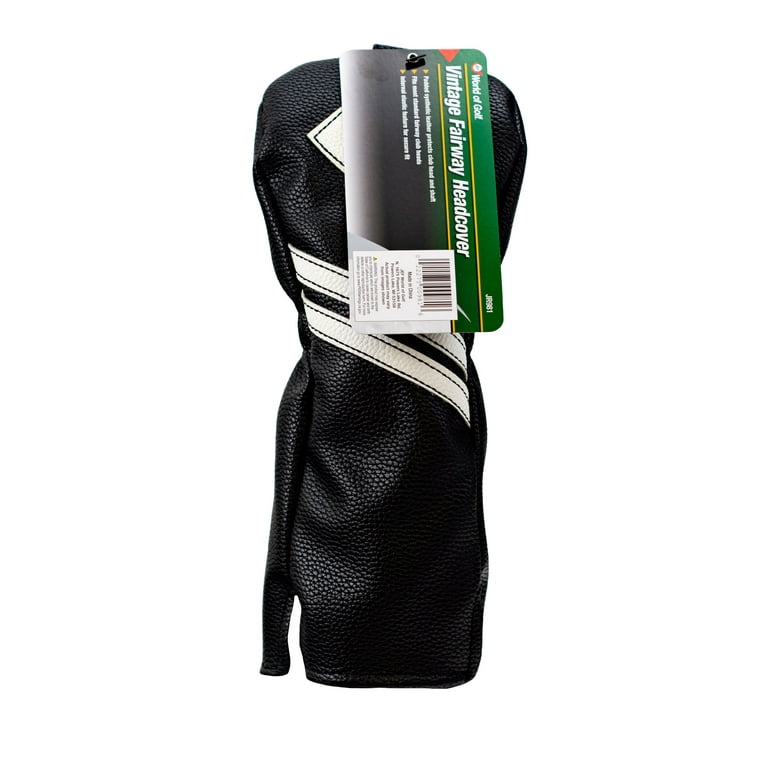The photograph displays a vintage Fairway golf club head cover designed to protect a club, likely a wood or driver. The head cover is constructed from a black, textured faux leather material and features distinctive diagonal white stripes running at a 45-degree angle. Attached to the cover is a green and black tag, which reads "World of Golf" and "Vintage Fairway head cover." The tag includes a barcode, though the model number is too small to discern. The background of the image is white, emphasizing the head cover’s design and the attached tag.